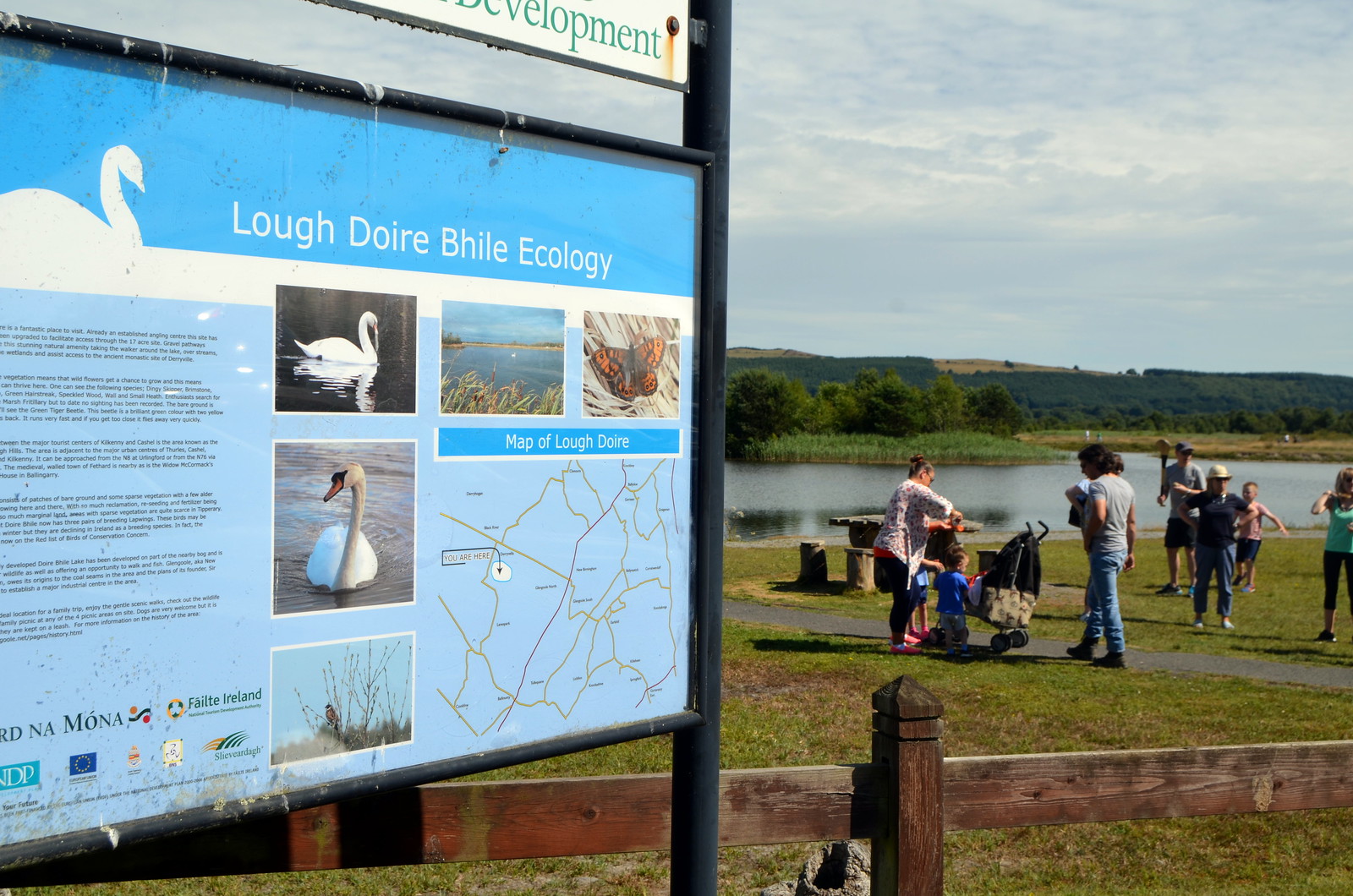This photograph, taken at an angle, portrays a bustling community park by a lake, central to the image, framed by a cloudy sky with layers of white and gray in the upper right. The background features scenic hills and lush trees. In the foreground on the right, a group of around ten people, some standing on a sidewalk and others on the grassy area, engage in various activities. Among them, a mom tends to a little boy in a black stroller, while a man in jeans and a t-shirt stands nearby. Another woman interacts with an infant beside a black baby carriage, and some individuals appear to be playing a catch game, possibly lacrosse.

On the left side of the image, a tall sign, standing on black poles, partially comes into view. The blue sign, decorated with a white outline of a swan at the upper left, announces "Lough Doire Bhile Ecology." The sign features text (some of which is cut off or too small to read), colorful pictures of swans on the lake, a monarch butterfly, and a large square map at the bottom. A wooden fence runs along the front of the lake, adding to the tranquil yet lively atmosphere of this ecological reserve. The vivid colors of the grassy area, the blue lake, and the varied attire of the visitors – including blue jeans, blue shirts, and white shirts – accentuate the vibrant community scene captured in this horizontally aligned rectangular picture.